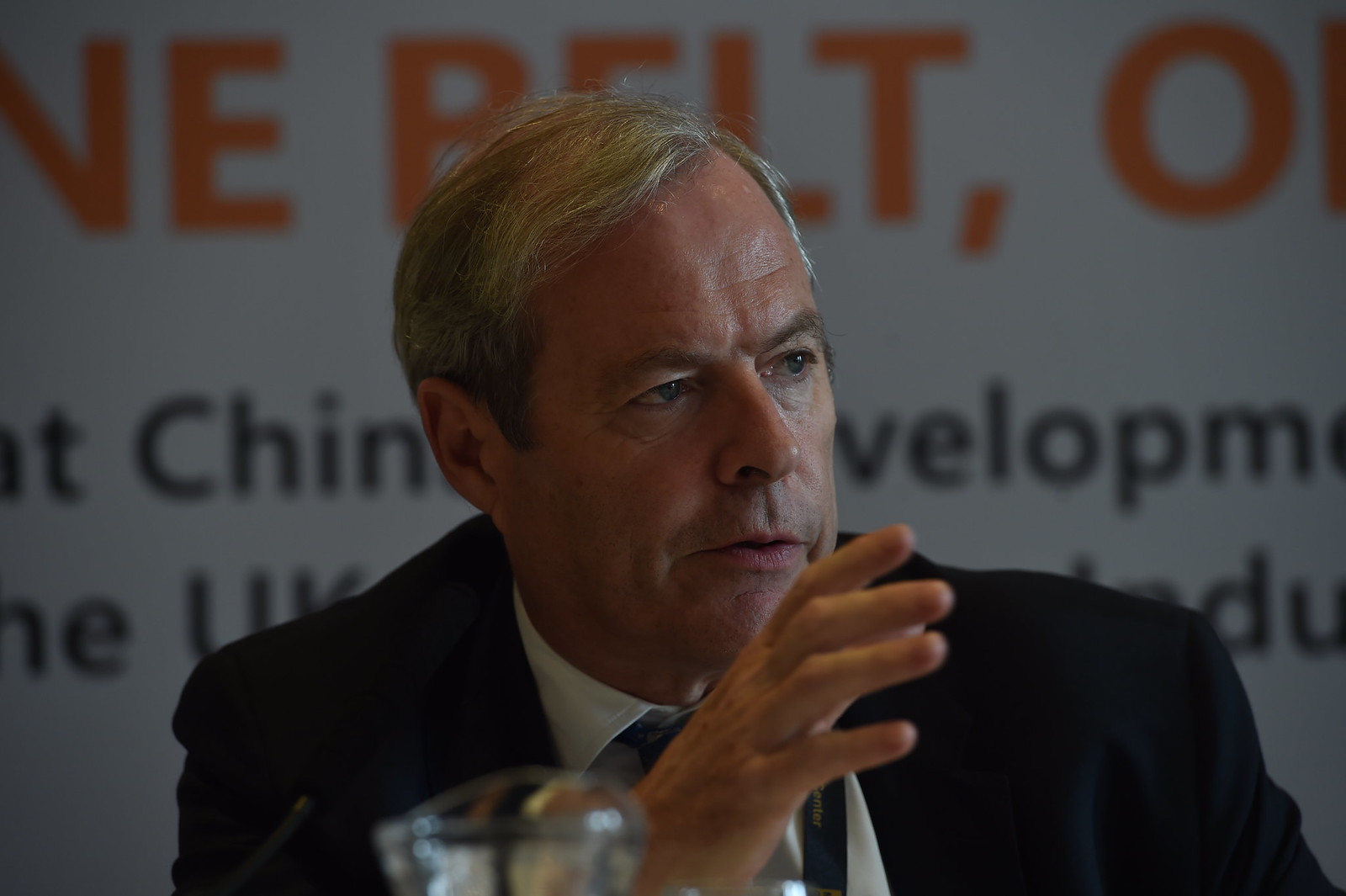The image features an older white male with a receding hairline and gray hair styled in a side part, possibly indicating that it was once darker. He is clean-shaven and has blue or blue-gray eyes. Dressed in a full black suit and tie, he appears to be speaking at an event, gesticulating with his right hand raised for emphasis, while he looks slightly to his left. His facial expression is neutral, conveying a stern or serious demeanor without appearing happy or upset. In the background, there's a large white backdrop with some orange text at the top and black text below it, partially readable with words like "China" and "development" visible. The event setting is further suggested by the zoomed-in view and fragmented text.